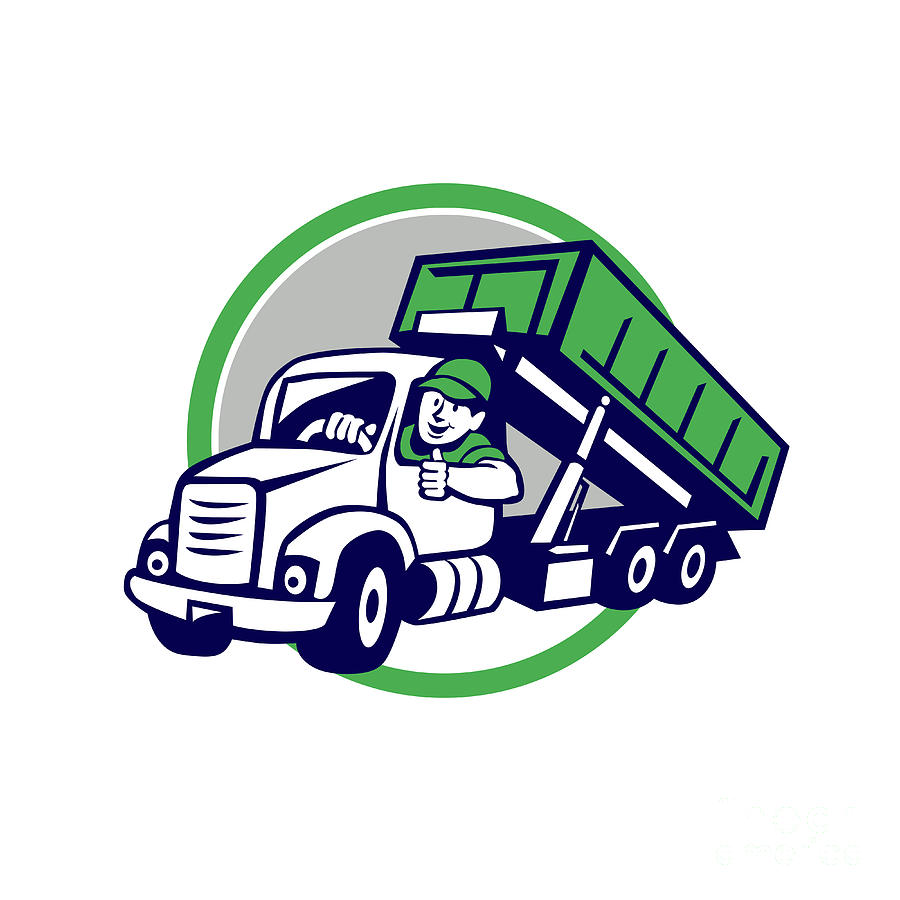This is a digital illustration depicting a cartoonish logo presumed to represent a delivery or waste removal company. The central element is a dump truck positioned as if about to dump its load. The truck features a green back dump section, while the cab is white, all outlined in deep navy blue. The driver, garbed in a green hat and shirt, humorously protrudes his head and arm out of the window, giving a thumbs-up with a cheerful smile. The truck is encircled by a prominent green rim, with the top half of the inner circle shaded gray and the bottom white, separated by a thin white border. The image, characterized by flat, shadowless colors, maintains a clean and captivating design, easily conveying a sense of service and reliability.